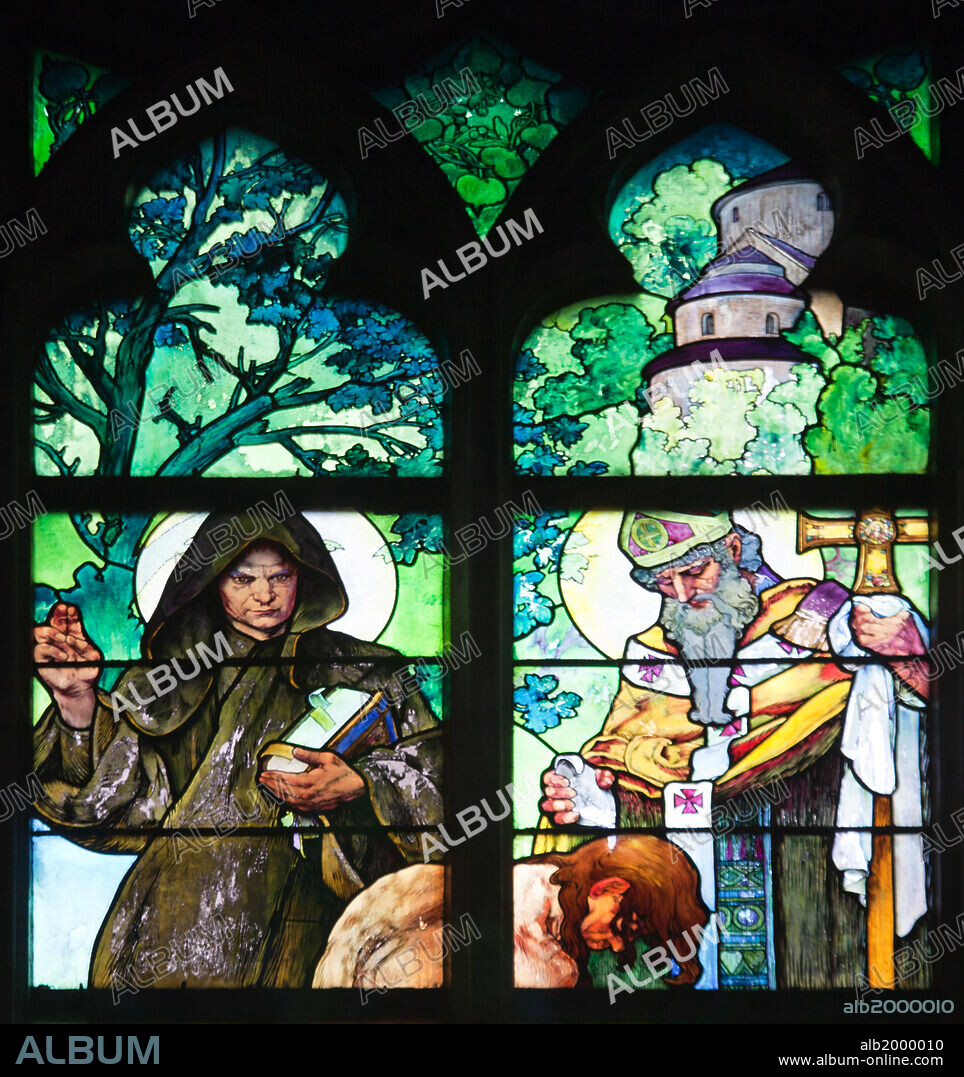This rectangular album cover, slightly taller than it is wide, mimics the look of a colorful stained glass window with intricate details throughout. The image features multiple elements: two dark-bordered, arched church windows divided by black bars, rich with predominantly green and blue hues. Watermarks with "album" in white or gray writing are scattered across the scene, along with an inscription at the bottom reading "www.album-online.com" and an encoded identifier "ALB20000010."

The windows display vibrant scenes of green foliage, with blue flowers on the right, and portray a serene outdoor setting with glimpses of a castle in the background. The windows' top edges are slightly clover-shaped, enhancing the ecclesiastical theme.

In the foreground of the left window stands a stern-looking monk dressed in a grayish-brown cape and hood, holding up his right hand and clutching a book in his left arm. The right window features a bishop, distinguished by a long white beard and ornate robes adorned with white ribbons, holding a cross and gazing down solemnly. Between these figures, in the center of the image, a shirtless man with his head bowed and hair falling forward kneels, his posture contemplative and subdued. 

Overall, the scene is a richly detailed, church-inspired mural capturing a moment of solemnity and religious reflection.